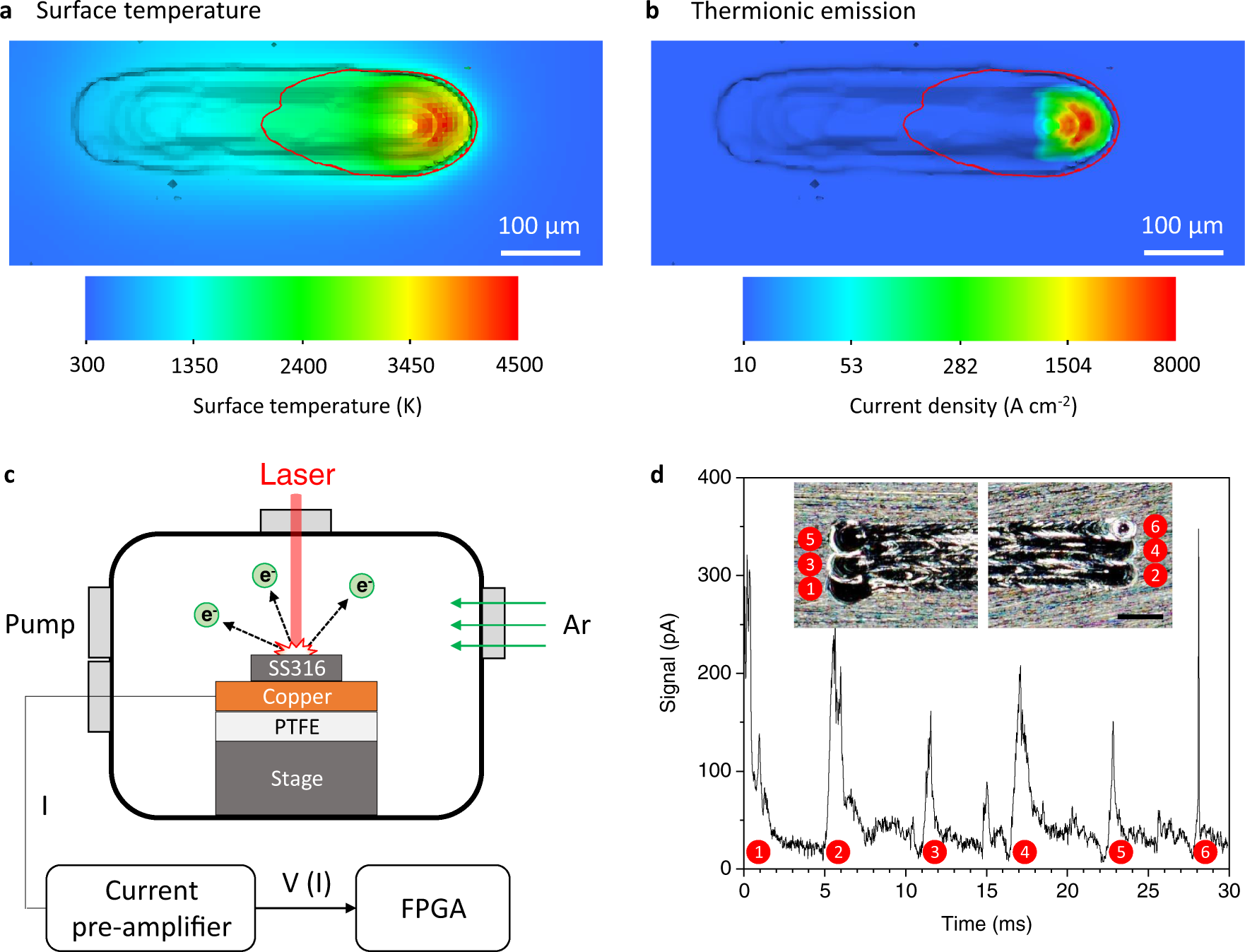The scientific diagram consists of four distinct parts. The top left image, labeled 'Surface Temperature,' displays a temperature map with a range from 300 to 4500, where the color gradient moves from dark blue representing cooler temperatures (300) to red indicating the highest temperatures (4500), transitioning through teal, green, yellow, and orange. To its right, labeled 'Thermionic Emission,' a similar map depicts density levels ranging from 10 (dark blue) to 8000 (dark red), highlighting regions of varying density. The third image, labeled 'C,' illustrates various stages of a process involving a laser, pump, copper, PTFE, SS316, and an amplifier. The fourth part, labeled 'D,' features a line graph showing the signal intensity over time, detailing the process dynamics.